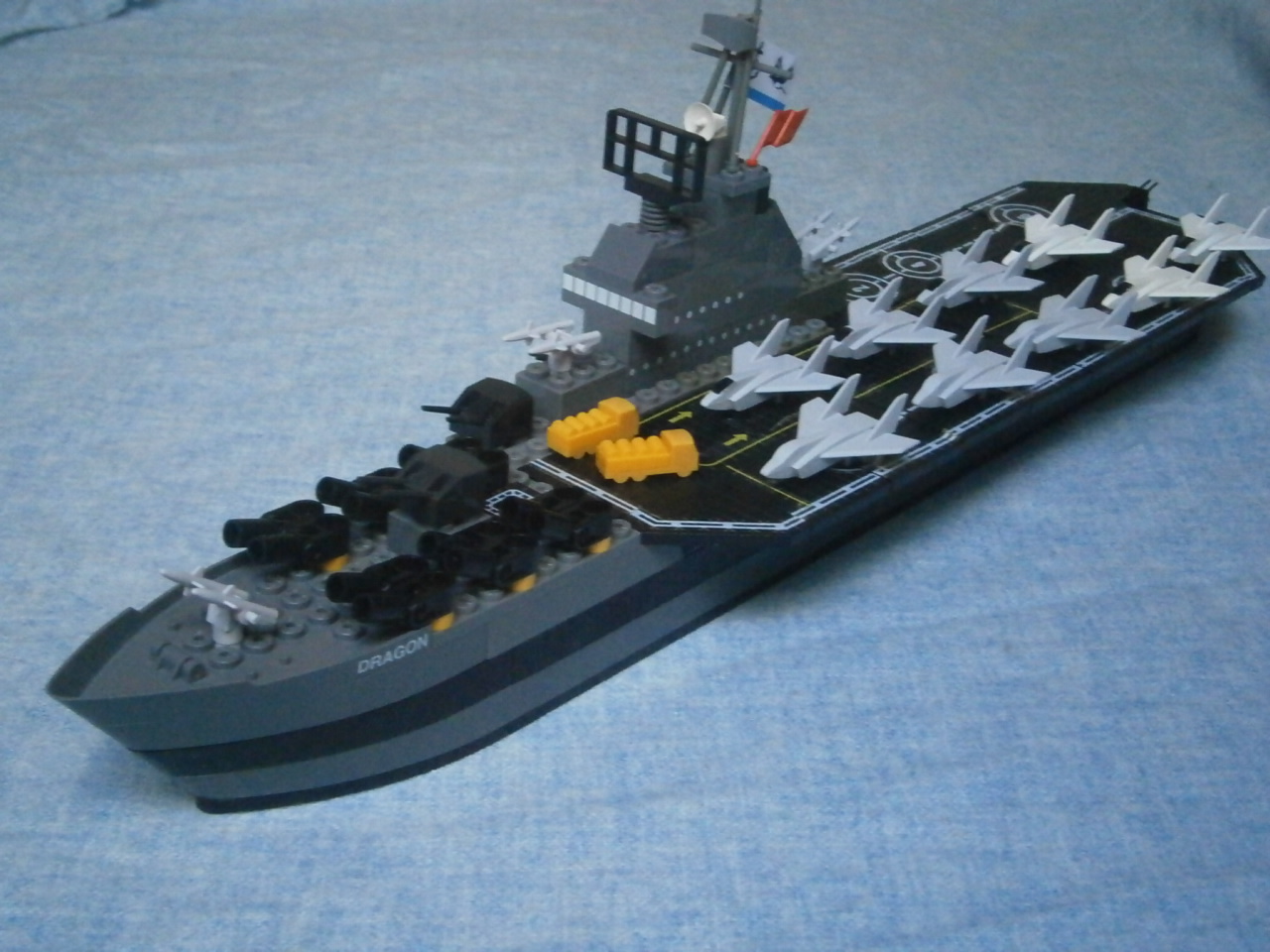The image features a detailed model of a gray Lego aircraft carrier named Dragon, positioned centrally on a grayish-blue fabric that mimics the appearance of water. The ship is angled, with the bow towards the bottom left and the stern at the top right. On the deck, there are nine white fighter jets, neatly parked on a black runway with distinctive yellow striping. Prominently placed at the front of the runway are two yellow Lego tanker trucks. The carrier is equipped with black cannons or armaments toward its bow and a black rotating radar atop the superstructure. The scene appears to be set indoors, creating a realistic miniaturized naval setting.